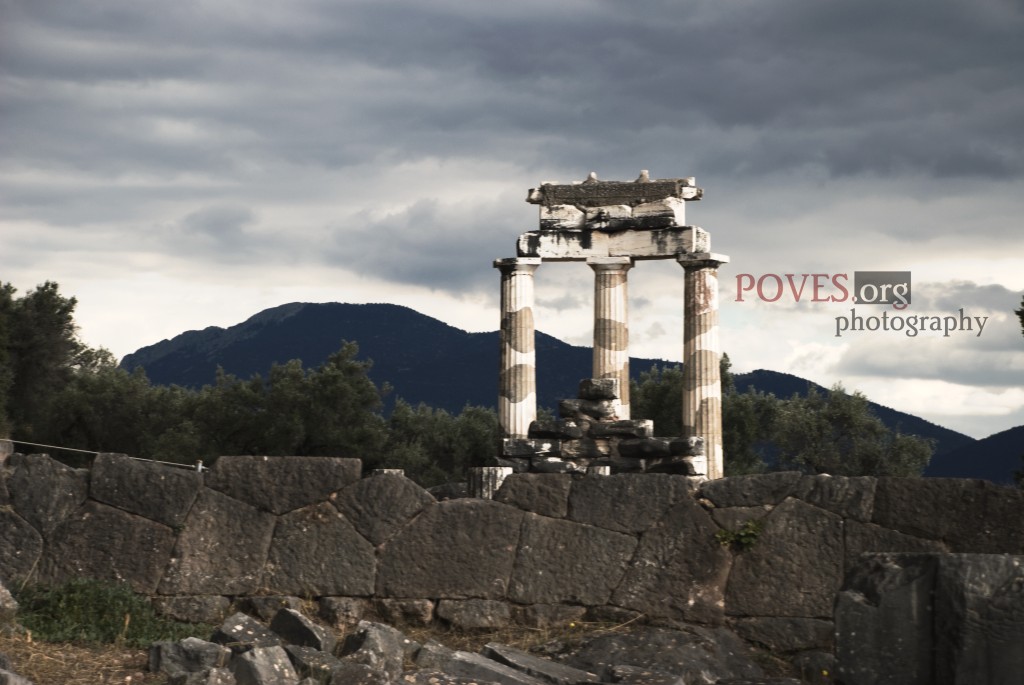The image depicts an eerie landscape dominated by an overcast sky filled with dark, wavy gray clouds tinged with bits of white. In the foreground, a dark gray stone wall, constructed from large, flat stone blocks, stretches horizontally. Beyond this stone wall, a trio of ancient white pillars, adorned with gray spots, stand tall and steadfast. Atop these columns rests a rectangular slab of matching white and gray stone, hinting at the remnants of a once-grand structure, possibly a Greek temple. Surrounding the scene are dark green leaves from nearby foliage, and in the background, a silhouette of a black mountain rises ominously. Clearly visible on the right side of the image, near the middle, is the text "POVES.org photography," marking the photograph's origin.